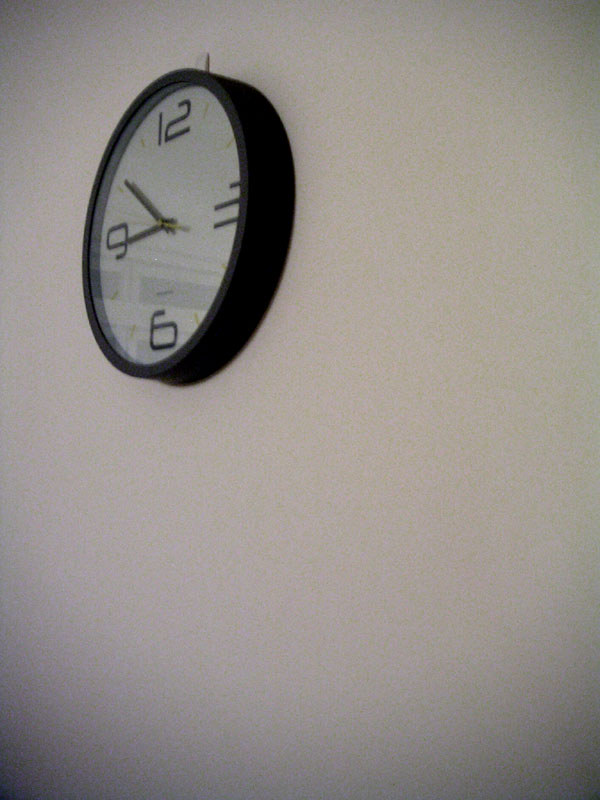This is a photograph of a modern wall clock hanging on a white, yet slightly dingy wall, possibly within an office setting. The clock is positioned at an angle, with the number nine further from the viewer and the number three closer. The clock's body is black with a reflective plastic cover, casting a small reflection likely from an opposite wall. The clock face is white, featuring black numbers and dashes: the 12, 3, 6, and 9 are prominently displayed in black, and the dashes representing the other hours are green. The time on the clock shows approximately 8:50, with the hour hand near the nine, the minute hand at the ten, and a gold second hand visible as it ticks around the face. The photograph is slightly out of focus and grainy, contributing to the overall dingy appearance of the wall color.